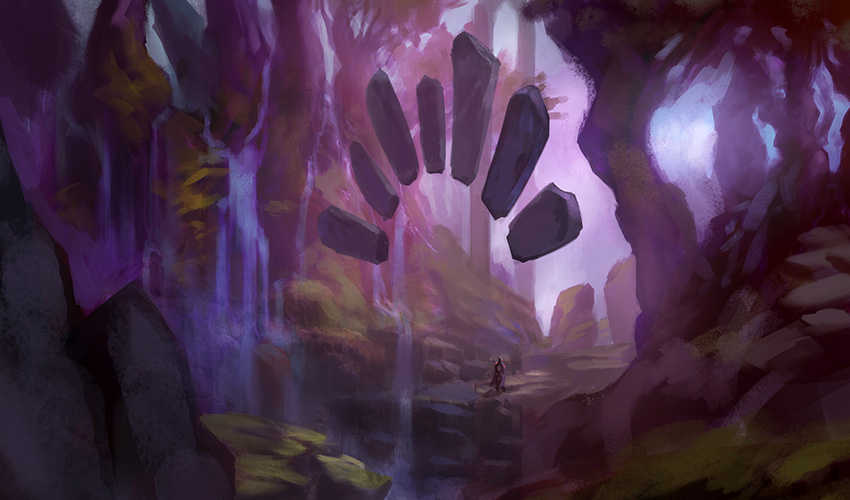The image presents a captivating, somewhat abstract, and artistic scene dominated by shades of purple. At the bottom center of the horizontally vertical composition, a tiny, indistinct figure stands on a flat section of rock. This figure is surrounded by an enchanting environment with numerous floating rocks—seven in total—that bear the shape and appearance of carefully carved tombstones.

On the left side of the image, a majestic waterfall cascades down over a series of rocks, adding a dynamic element to the serene surroundings. The scene is set against a backdrop of towering trees and sprawling boulders that seem to converge towards what could be interpreted as a mystical entryway or castle area. Above, in the upper right-hand corner, a patch of blue sky peeks through, contrasting with the primarily purple and gray hues of the landscape.

The overall ambiance of the image is whimsical and otherworldly, suggesting a scene from an animated series or a fantastical book, imbued with a sense of magic and wonder. The combination of natural elements and the ethereal details evoke a dreamlike quality, making it a mesmerizing piece of art.